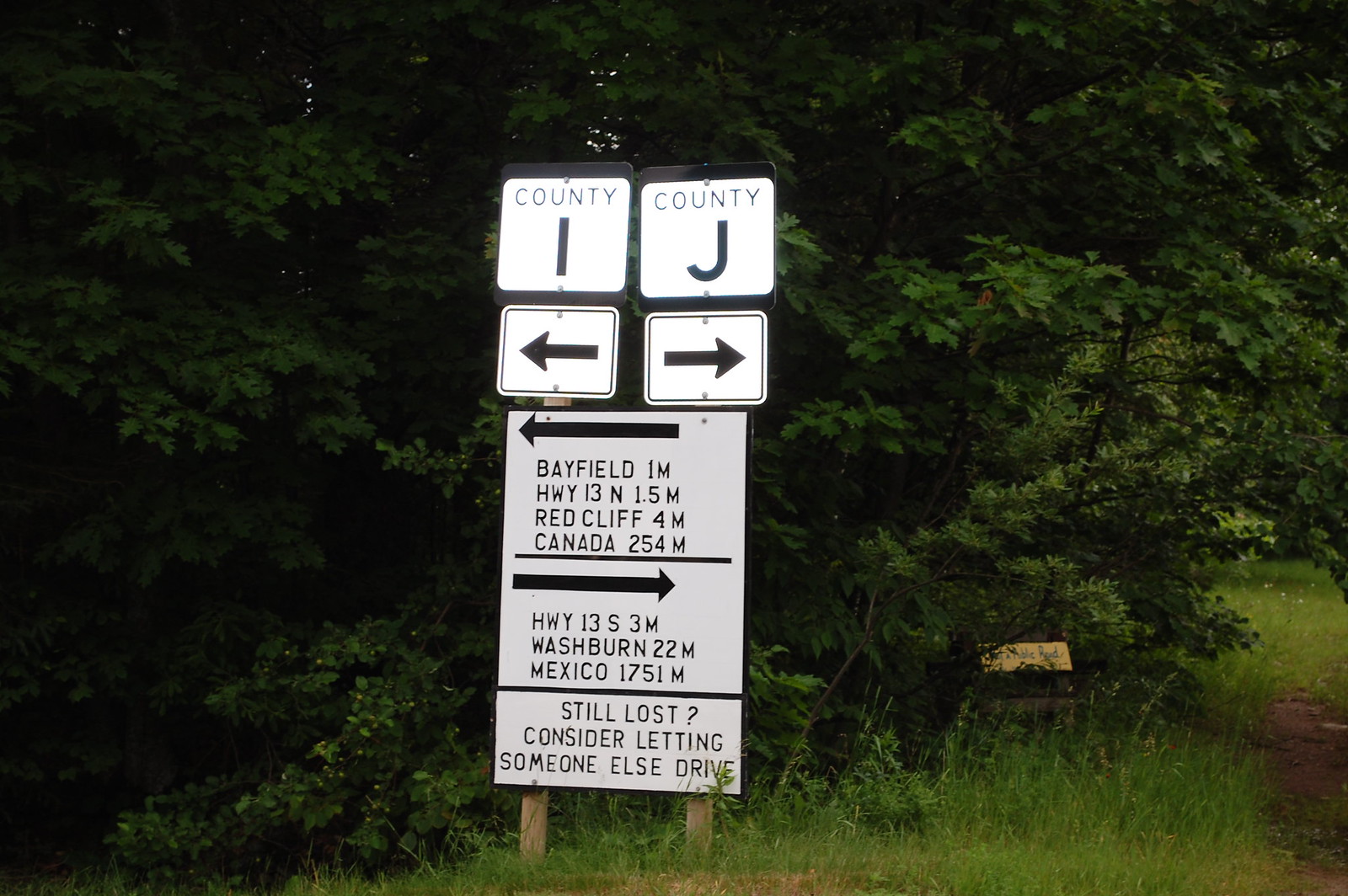A detailed road sign sequence mounted on two wooden posts stands prominently against a backdrop of lush trees and green grass. At the very top of this assembly, two white square signs indicate directional guidance for County I and County J: the left sign reads "County I" with an arrow pointing left, and the right sign reads "County J" with an arrow pointing right. Below this, a detailed set of directions is provided. An arrow pointing left informs travelers that Bayfield is 1 mile away, Highway 13 North is 1.5 miles away, Red Cliff is 4 miles away, and Canada is 254 miles distant. 

An arrow pointing right directs travelers towards Highway 13 South, located 3 miles away, with Washburn at 22 miles and Mexico at an astonishing 1,751 miles. A humorous sign at the bottom reads, "Still Lost? Consider Letting Someone Else Drive." The entire signpost is nestled in a serene, wooded area with abundant trees and verdant grass surrounding it, adding to the scenic and somewhat whimsical nature of the location.